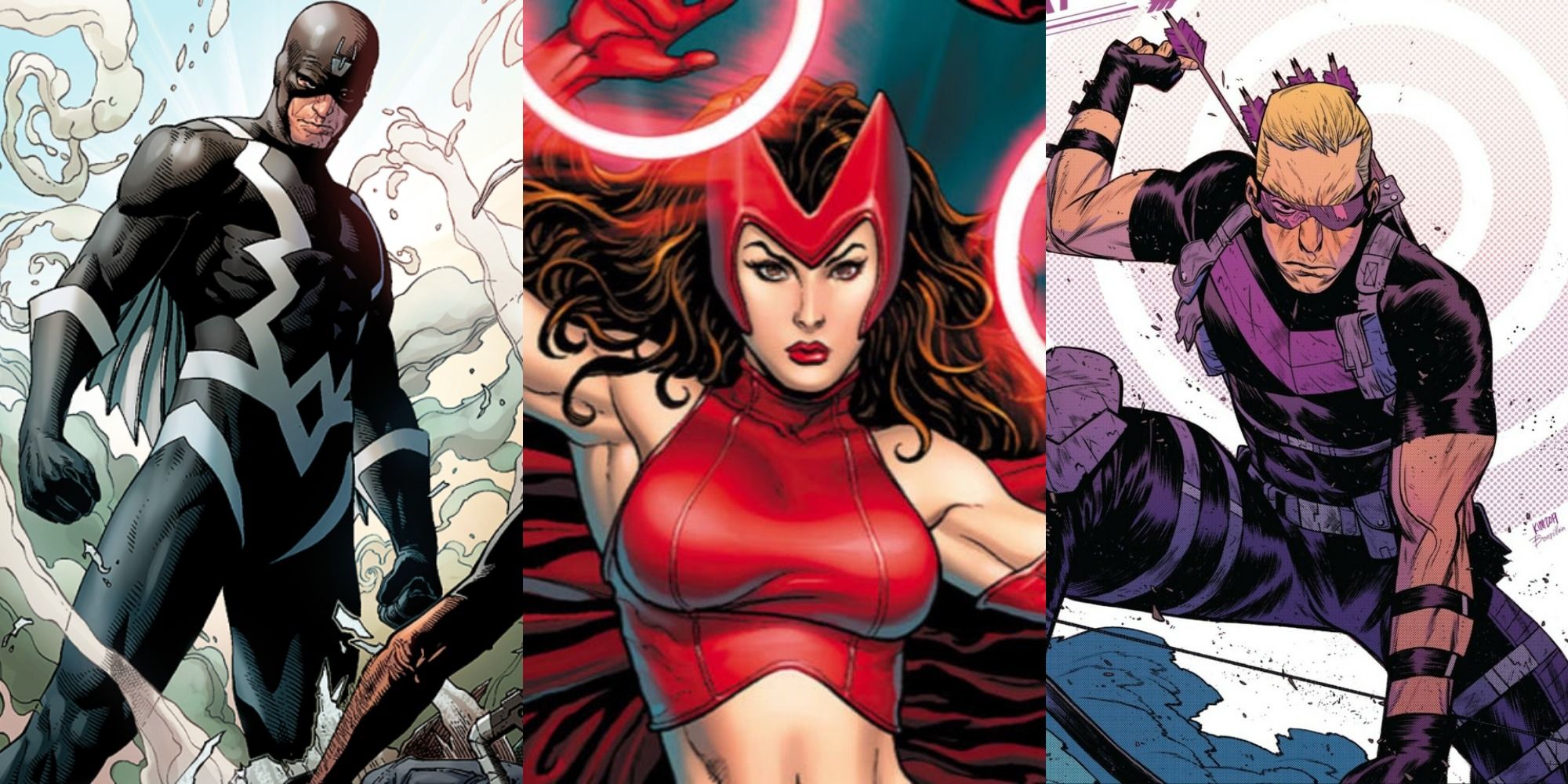The image is a collage of three comic book characters, each occupying a third of the rectangular frame, which has a width three times its height. Starting on the left, the first character is a muscular superhero dressed in a skin-tight black suit that covers every inch of his body except his mouth and nose. The suit is detailed with white zigzag lines and has white accents on the edges of his gloves. He is standing with his arms by his sides, hands clenched into fists, surrounded by plumes of smoke and dust, giving the impression of a dynamic action scene.

The character in the center is a woman wearing a red, sleeveless crop top made of leather, exposing her midriff. She sports a red crown or helmet that covers her forehead and ears but leaves her eyes, nose, and mouth visible. Her long brunette hair cascades down to her shoulders, and she has red lipstick. Her hands are outstretched, and red glowing lights encircle them, set against a blue background.

The character on the right is a man in a tight, purple outfit, crouched down with one hand on the ground and the other reaching back for an arrow from the quiver on his back. His outfit includes black leather pants and a purple chest piece, as well as purple goggles or sunglasses. He has blonde, slicked-back hair and a determined scowl on his face. The background behind him is white with smoke and some circular patterns, hinting at another intense action moment.